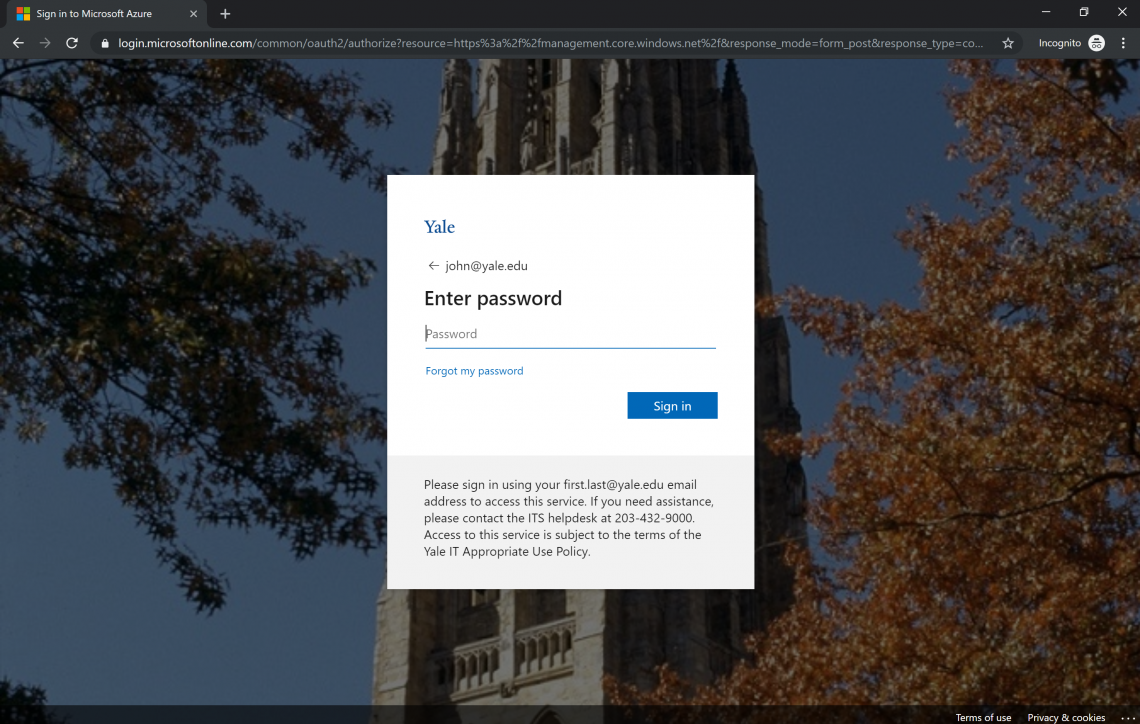The image captures a Microsoft Azure sign-in screen at the URL "login.microsoft.com/oauth2/authorize?" The URL includes various parameters like resource, response mode, and response type.

The background of the image features a scenic landscape with trees on both sides, adorned with golden leaves that appear crisp, possibly indicating autumn. A majestic stone tower with a spiral structure stands prominently in the background, adding a touch of grandeur to the scene.

At the center of the image is the sign-in interface with a splash screen. In blue text, "Yale" is prominently displayed, and beneath it, the email address "john@yale.edu" is shown. Below that in black text, instructions are given to "Enter password," with options for "Forgot my password" and a blue "Sign in" button.

Additional text advises users to sign in using their "first.last@yale.edu" email address for access to the service. For assistance, users are directed to contact the ITS helpdesk at 203-432-9000. It also mentions that access to the service is subject to Yale's ITS appropriate use policy.

In the bottom-right corner, there is a note for "Privacy and Cookies," providing further information about data usage and privacy policies.